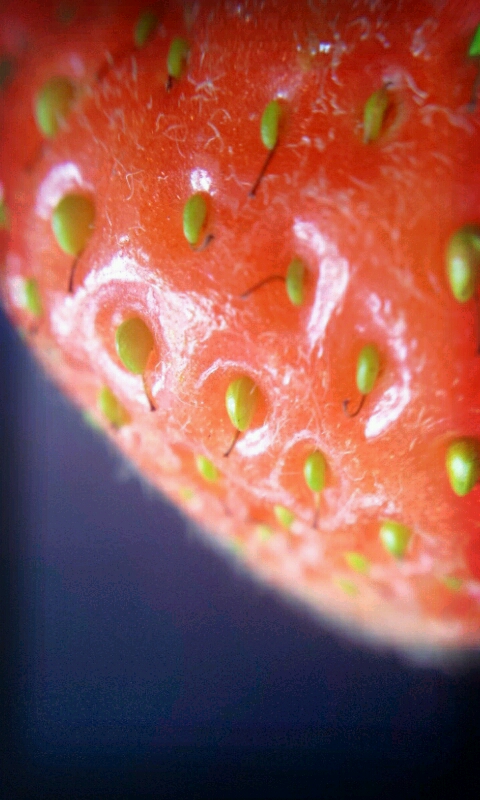This close-up photograph features the flesh of a large, reddish-pink fruit, or possibly another type of seed-bearing plant, set against a navy blue background. The focal point reveals several glossy, green seeds or beans protruding halfway from pits within the vibrant red-pink flesh. These seeds, some with straighter, others with curlier stems, vary in their embedment; some are more deeply tucked into the plant, while others extend out quite far. The seeds present a shiny appearance, matching the lustrous look of the fruit itself. The shot captures a slightly blurred background, indicating a focus on the foreground elements and giving the viewer a side perspective of the intriguing organic subject.